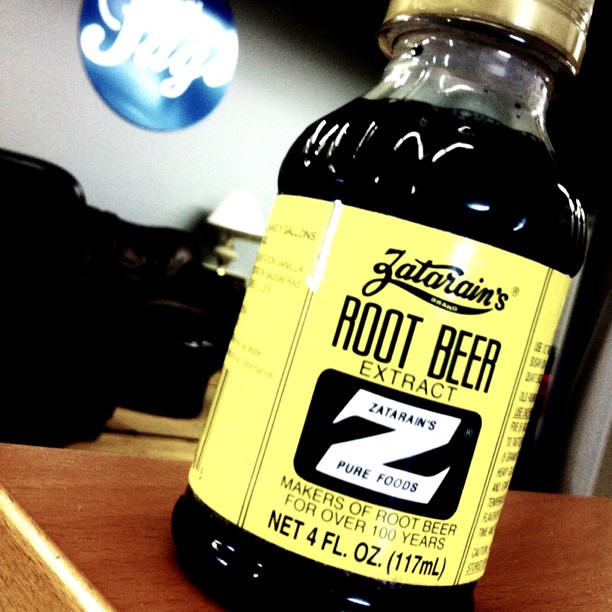The image is a close-up, diagonally-tilted photograph of a small, dark bottle of Zatarain's Root Beer Extract. The bottle has a golden cap and is made of either glass or plastic, with light reflecting off its surface, making it appear quite shiny. The label is light yellow with black text, prominently featuring the Zatarain's logo in a stylized script. It states “Zatarain's Root Beer Extract” and includes a black rectangle with a white "Z" in the middle, indicating "Zatarain's Pure Foods." Additional text on the label reads, “Makers of Root Beer for over 100 years” with “Net 4 FL. OZ. (117 mL)” below it. The background contains a wooden table, with indistinct furniture and possibly a desk lamp, and a white wall. The contents of the bottle are very dark, almost black.